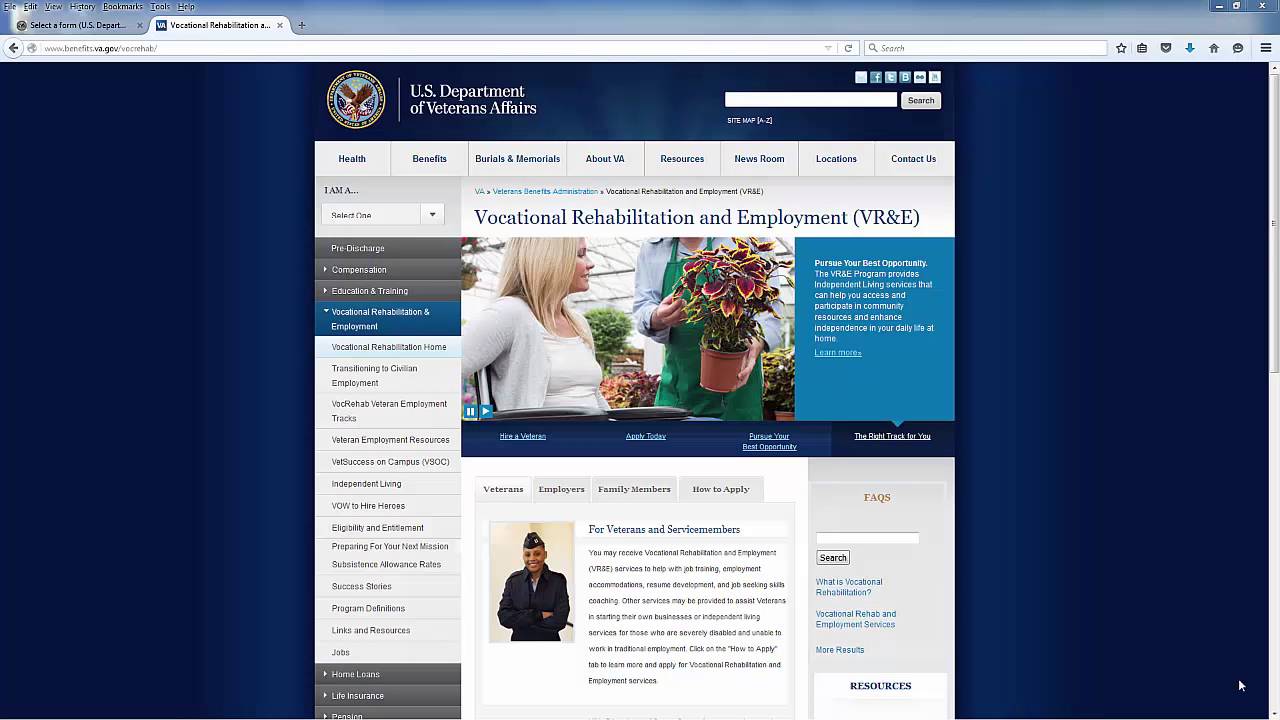The image displays a web browser with two open tabs. The visible tab is focused on the US Department of Veterans Affairs website, while the other tab titled "Selective Form, US Department" is not active.

The US Department of Veterans Affairs webpage is prominently featured in the center, flanked by dark blue margins on both sides. In the top right corner, there are links to various social media platforms, including Facebook. Directly below these links is a white search box accompanied by a grey search button for entering and executing search queries.

The main logo of the site is positioned to the left of the search box, depicting a hawk landing within a circle, with the text "US Department of Veterans Affairs" to its right. Beneath this logo, a grey banner spans the page, displaying a series of headings: "Health Benefits," "Burials and Memorials," "About Us," "Resources," "Use Room," "Vocations," and "Contact Us."

On the left-hand side of the page, there is a vertical menu with a series of options that are somewhat difficult to read due to the font. The active selection is "Vocational Rehabilitation and Employment (VR&E)," denoting that the page's content currently pertains to this topic. Below, various images and blocks of text provide further information about vocational rehabilitation and employment services.